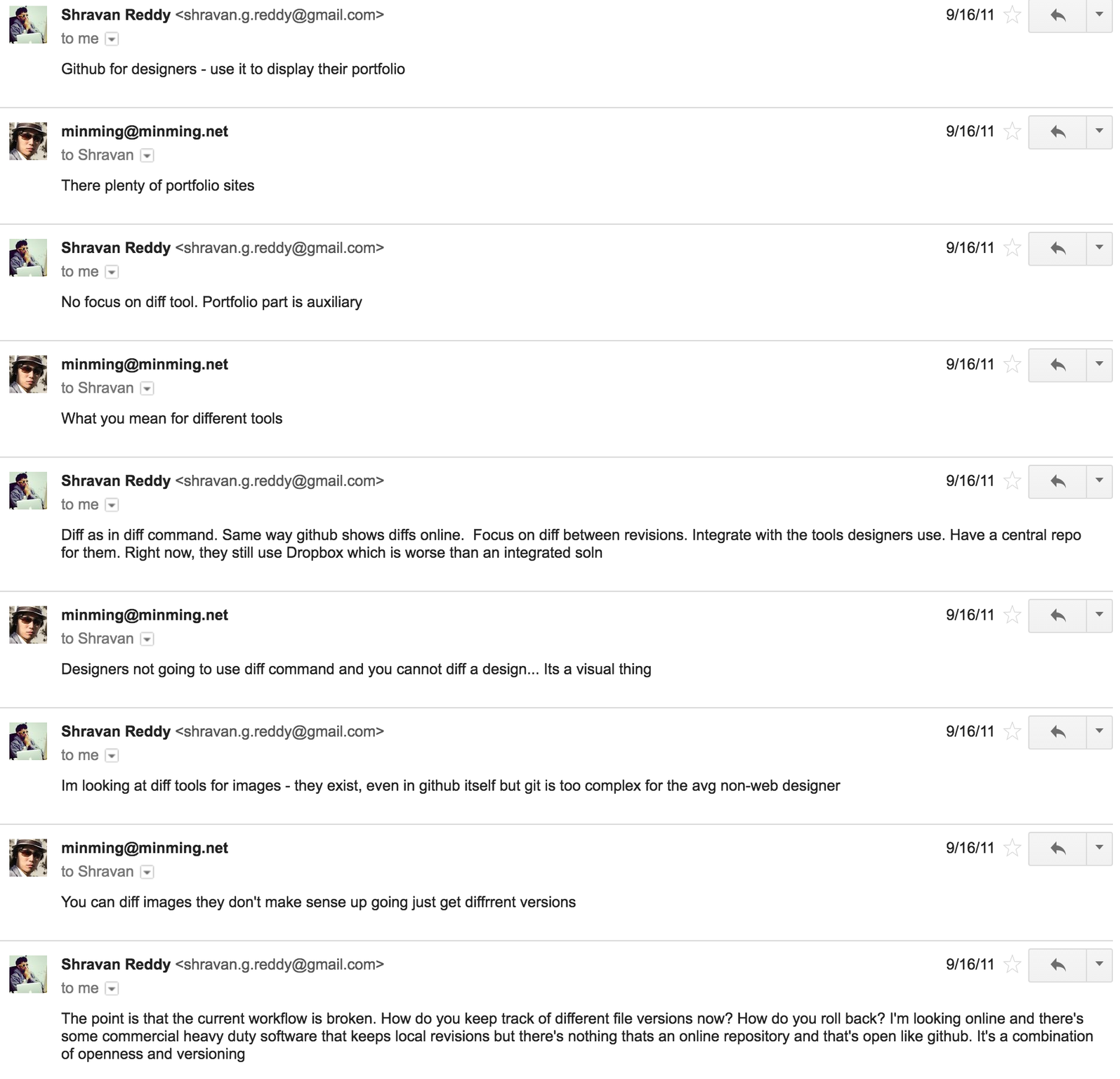The image displays a portion of a website that profiles individuals, likely on a professional platform. The page is laid out in fine print and features small portrait photos of nine different individuals on the left-hand side. Each profile consists of a name, a short description, an email address, and possibly other personal information. 

In the middle section, there appears to be a conversation between two individuals, Chevron Ready, whose email is chevronready@gmail.com, and Min Ming, associated with minming.net. They discuss the utility of a GitHub-like platform for designers to display portfolios with a focus on a "diff tool," which highlights differences in designs similarly to how GitHub shows changes in code. Chevron emphasizes the importance of integrating tools that designers already use and creating a central repository, as opposed to using services like Dropbox, which they find less efficient.

On the right-hand side of the page, there are two columns and a date displayed as 9-16-11. There are also navigation options allowing users to go back or choose other actions within the site.